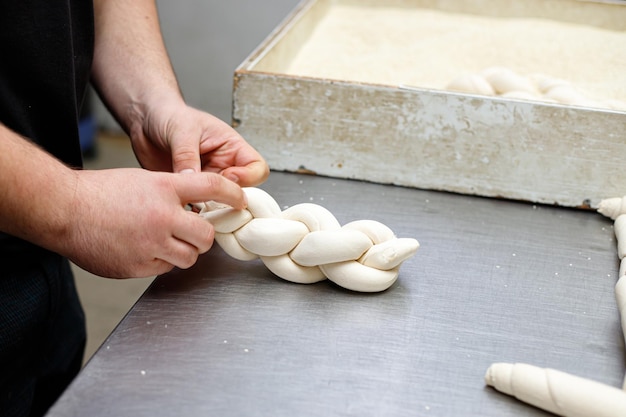In this detailed photograph, a male chef with Caucasian features is meticulously braiding three long strands of dough into a thick rope atop a stainless steel surface. His fingertips delicately pinch the end of the braid, ensuring it holds together. In the background, a square wooden container filled with flour contains another completed braid, suggesting preparation for baking. Other rolled dough pieces, likely destined to be braided next, rest in the bottom right corner of the image. The scene hints at the preparation of challah bread, a traditional bread in Jewish culture. The chef's focused hands, marked by the presence of arm hair and a lack of nail polish, indicate experienced craftsmanship in the art of bread-making.